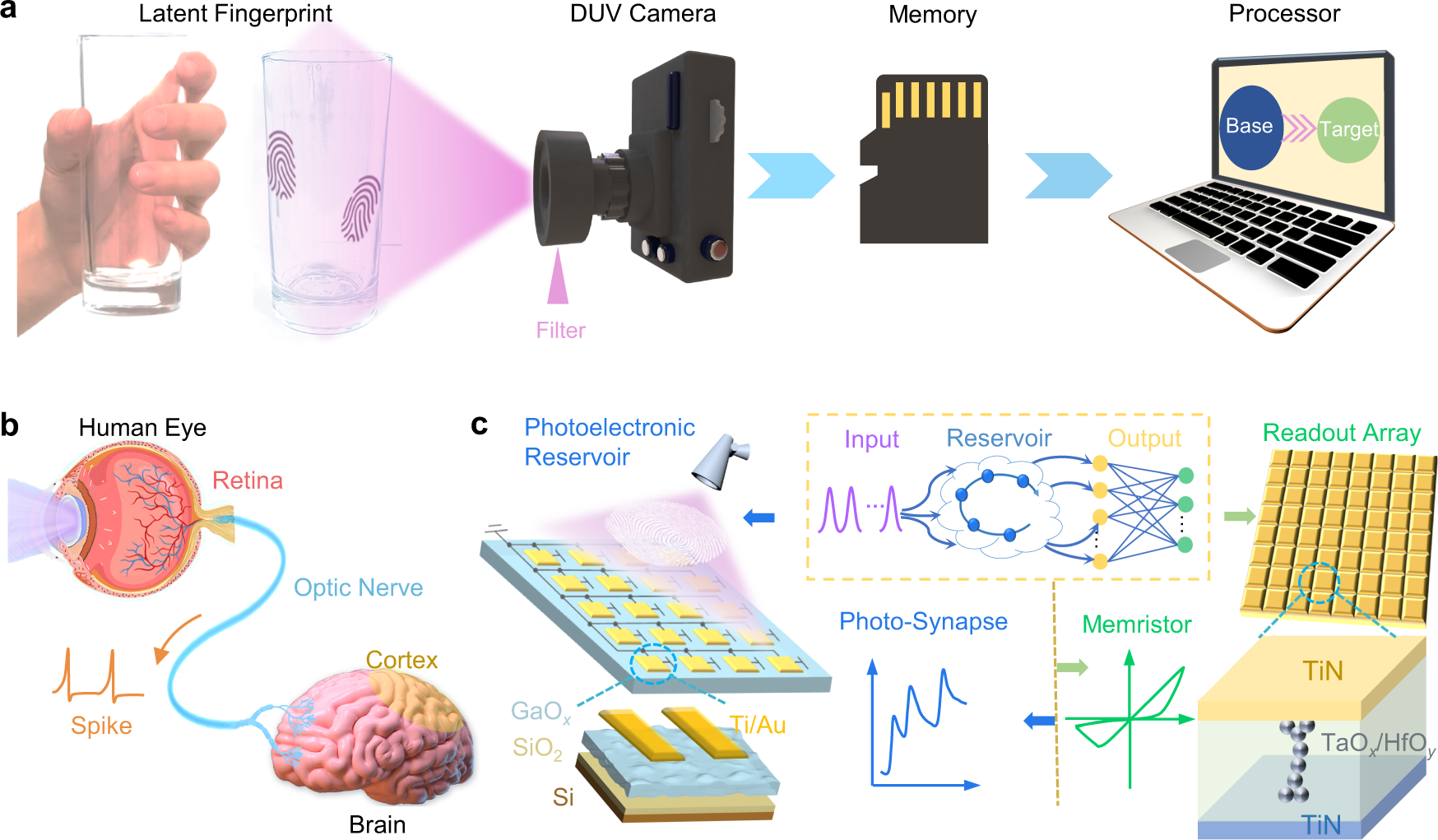The diagram is divided into three labeled sections: A, B, and C. Section A occupies the entire top level and illustrates the process of latent fingerprint collection and processing. It features five images: the first two show a person holding a glass with two fingerprints, captioned "latent fingerprint." Next is an image labeled "DUV camera," indicating the use of a camera with a deep ultraviolet filter to capture the fingerprint. Following this, a flowchart illustrates the transfer of fingerprint data to memory (depicted by a memory card) and then to a processor (represented by a computer).

Section B, located at the bottom left, focuses on the human visual system. It includes drawings of the human eye and brain with a flowchart linking the retina, optic nerve, and cortex, detailing the visual processing route from the eye to the brain.

Section C, found at the bottom right, details a photoelectric reservoir system. It includes several drawings of components such as a light shining on a rectangular sensor, labeled with various chemical compounds like GAO2, SIO2, S, TIAU, and arrays like the "readout array" and "photo synapse." The diagram indicates input and output processes and references to memory storage, suggesting the portrayal of a semiconductor-like device.